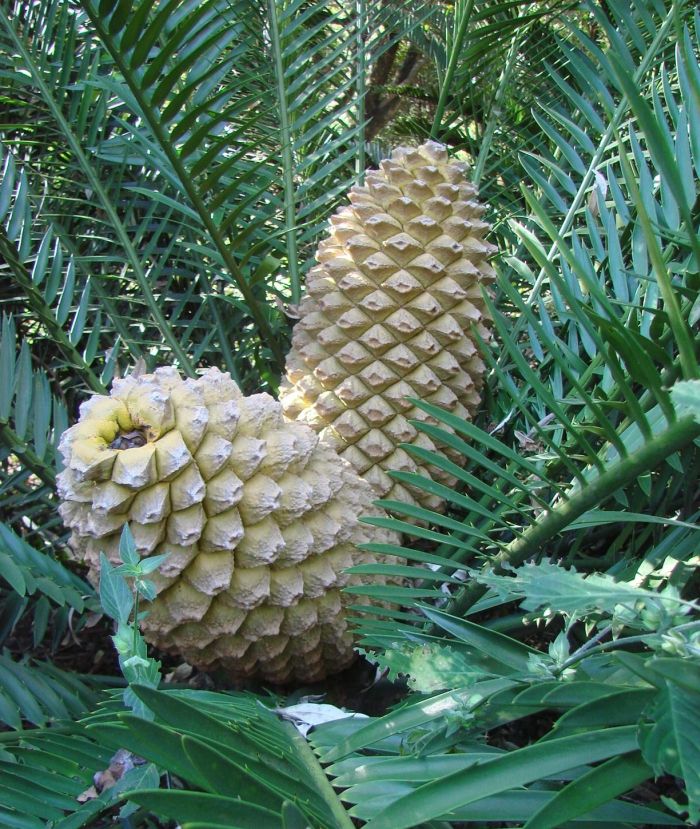The image features an outdoor, daytime view of a pineapple plant, set against a backdrop likely indicative of a jungle or forest environment. Central to the composition are two prominent pineapple fruits, which are long, oblong, and characterized by their brown, textured skin adorned with multiple diamond-shaped spikes. The pineapples display a hint of yellow coloring and white-tipped points on their ridges, with the left fruit featuring a distinct brown center at the top. Surrounding the fruits are lush, green leaves that have a fern-like appearance, extending out from the base of the plant. These thick, sturdy leaves fan outwards and are edged with pointed tips, providing a striking contrast to the textured pineapples in the center. The overall color palette includes various shades of green, light brown, beige, and some black accents, adding depth and vibrancy to the natural scene. The fruits are positioned such that one leans towards the bottom left of the image while the other points upwards, illustrating the natural, ungroomed growth of the plant.